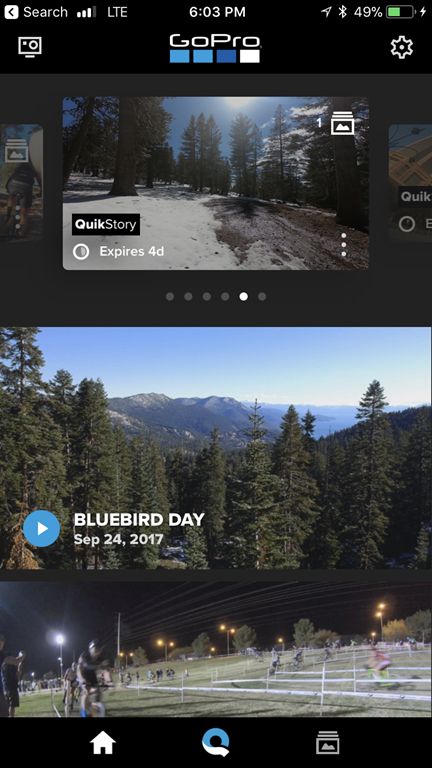This image showcases a GoPro app interface on a smartphone, likely an iPhone, given the layout. At the top, the GoPro logo is prominently displayed, transitioning from dark blue to white, with the time, battery percentage, and cell phone signal strength visible, indicating it's a mobile app. The top-right corner has a settings button, while the top-left corner appears to feature a display image setting button. 

Below this header, the main content area displays a series of old photos taken with a GoPro in 2017. One notable image features a serene scene with trees on a clear day captioned "Bluebird Day, September 24th, 2017." 

Further down, there are nighttime images of people enjoying a game, possibly involving bicycles. At the bottom, there are three main navigation buttons: a home page icon, a central button likely used for activating the GoPro camera, and an images section icon for accessing additional photos.

This detailed layout captures the essence of the GoPro app's interface, providing a functional and user-friendly experience for managing and viewing photos and videos taken with a GoPro camera.